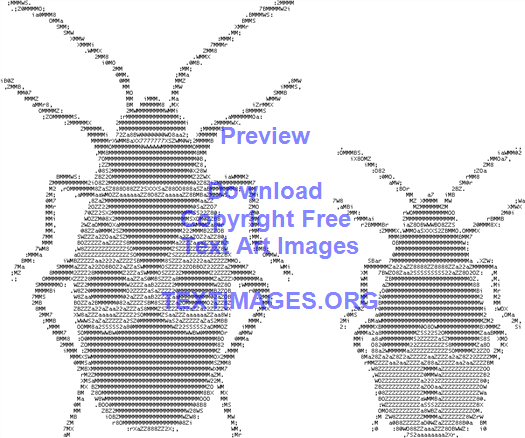Set against a crisp white background without any borders, the image showcases two intricate figures resembling cockroaches, crafted entirely from typewriter text characters. On the left, a larger, more complex cockroach features a composition of black and gray letters, numbers, and symbols. It boasts eight legs in total, with four on each side, and displays a pair of prominent wings that resemble teardrops with circular details. To the right, a smaller cockroach, approximately half the size of its counterpart, mirrors this artistic style with similar text characters and wing shapes. Both figures appear to be crawling across the page. Superimposed in a striking blue font, the text reads: "Preview. Download copyright-free text art images," and directs viewers to textimages.org, with the website URL displayed in bold, all-capital letters.